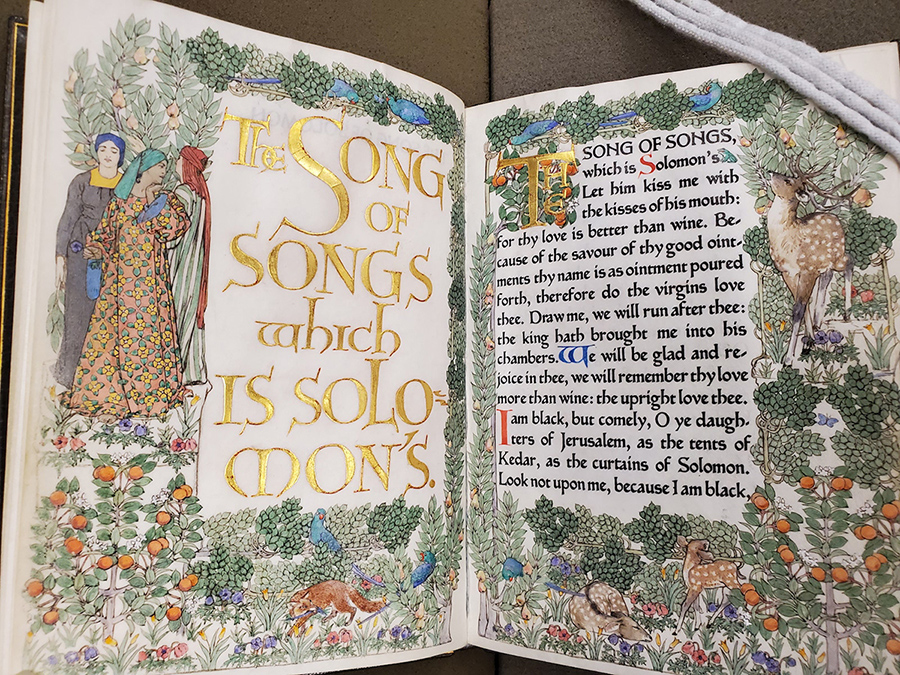The image depicts an open book richly adorned with illustrations and detailed text. On the left page, there is a vibrant illustration featuring three women adorned in colorful robes and headdresses; the woman on the left dons a dark gray robe with a yellow neckline and a blue headdress, the middle woman wears a yellow floral design against an orange background with a green headdress, and the woman on the right sports a white and green striped robe with a red headdress. Surrounding these figures are lush drawings of peach trees, various birds, animals, and flowers. Prominently displayed in the center of the left page is the title "The Song of Songs, which is Solomon's" inscribed in large gold letters.

The right page mirrors the intricate foliage and fauna of the left, depicting peach trees, deer, birds, and exuberant floral designs, but notably lacks the human figures. At the top left corner of this page, "The Song of Songs" is again highlighted in gold, with a large decorative 'T' as part of the word "The." Below, a block of text unfolds, commencing with "The song of songs, which is Solomon's," and continuing with a passage from the biblical text: "Let him kiss me with the kisses of his mouth, for thy love is better than wine. Because of the savor of thy good ointments thy name is as ointment poured forth; therefore do the virgins love thee. Draw me, we will run after thee; the king hath brought me into his chambers; we will be glad and rejoice in thee. We will remember thy love more than wine; the upright love thee. I am black, but comely, O ye daughters of Jerusalem, as the tents of Kedar, as the curtains of Solomon. Look not upon me, because I am black."

Adding to the charm of the page on the right, three delicate white ropes rest at the top edge, highlighting the blend of elegance and intricate craftsmanship in this illustrative and textual composition.